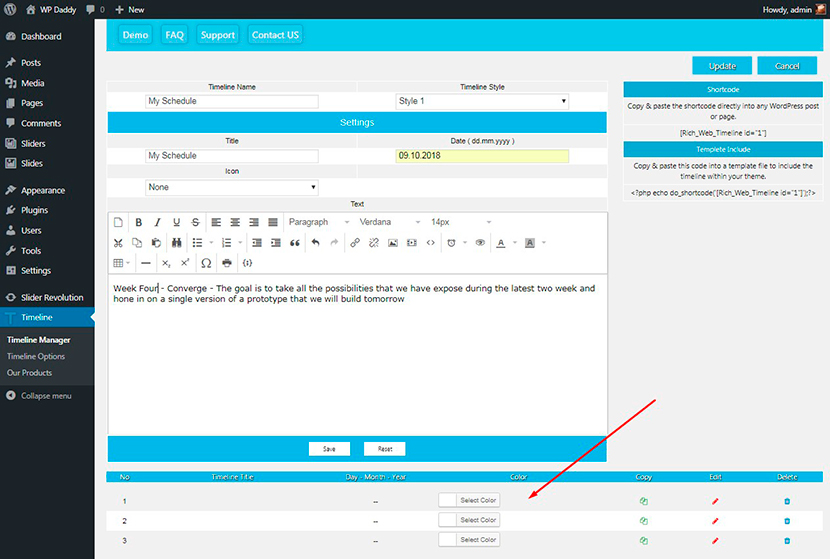A screenshot of a website interface prominently displays a black sidebar on the left containing various navigational icons with corresponding labels such as Dashboard, Posts, Media, Pages, Comments, Sliders, Slides, Appearance, Plugins, Users, Tools, Settings, Sticker, Resolution, Timeline, Timeline Manager, Timeline Options, and Our Products. The 'Timeline' option has been selected, highlighted in blue against the dark background.

The main content area, after selecting 'Timeline,' features fields titled 'Timeline Name' and 'Timeline Style'. The current style is 'Style 1', selectable via a dropdown menu. A blue, elongated rectangular button labeled 'Settings' is visible. Below this, there are entries for 'Title' and 'My Schedule'. A date field is filled in with '09/10/2018'. Further down, a text field contains a goal statement: "The goal is to take all the possibilities that we have exposed during the latest two weeks and home in on a single version of a prototype that we will build tomorrow."